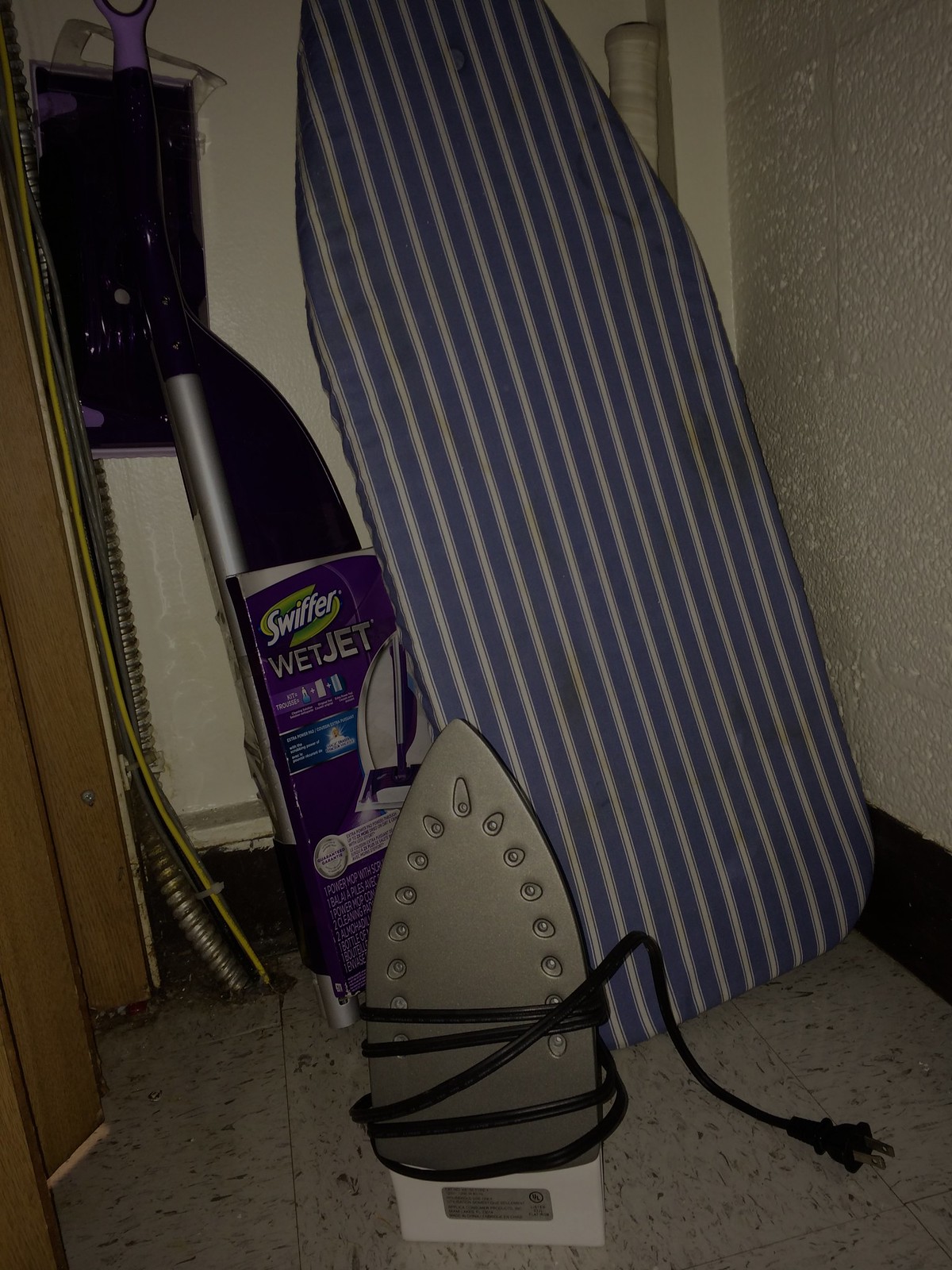This detailed image captures the inside of a small utility cupboard, perhaps located under the stairs. The walls are white and textured, possibly wallpapered, and there is a black skirting board at the base. The floor features industrial-looking tiles. Centered prominently at the bottom of the image is an iron, standing upright on the floor with its cord wrapped around it and an American plug lying off to the side. Despite its placement, the iron appears unused. Behind it, there's a Swiffer WetJet, still in its packaging, indicating it's for cleaning floors. To the side, we see a wide ironing board with a well-fitted cover featuring horizontal stripes in navy blue and white, giving it a nautical feel. The cupboard also has visible metal-shielded wiring running down the wall, enhancing the room’s utilitarian aspect, and the overall image is taken in low light.